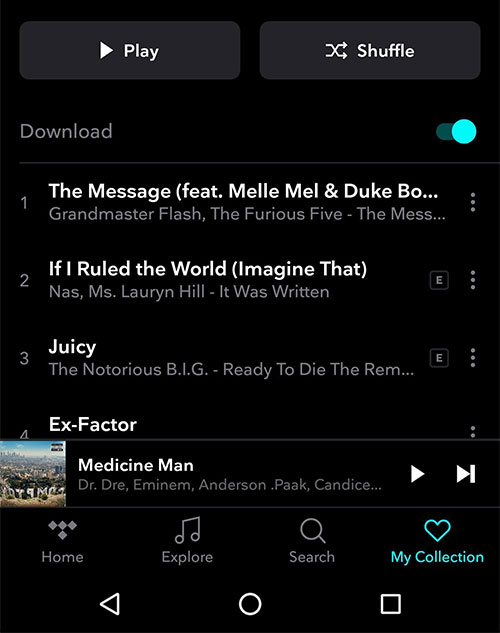The screenshot displays a music streaming interface, likely on a mobile device, featuring a list of four songs. The interface closely resembles that of Spotify or a similar music application. At the top of the screen are two side-by-side buttons. The left button, labeled "Play," features a triangle icon, while the right button, labeled "Shuffle," displays a shuffle icon. Both buttons use a bold, white, sans-serif font with capitalized first letters.

Directly below these buttons, the word "Download" appears in slightly larger gray text in a sans-serif font. On the same line, a toggle button on the far right is turned on, indicating that all four songs are being downloaded.

The four visible songs each display the song title in bold white sans-serif text, with the artist's name beneath it in smaller, non-bolded gray text. To the right of each song title, a set of three gray dots suggests an additional menu for further options.

At the very bottom of the screen, a currently playing song is indicated within a small bar. The song title appears in bold, with the artist's name beneath it in gray and not bolded. This bar also includes two icons: a play/pause icon and a next track icon. Below this, there's another menu, though its details are not specified in the description.